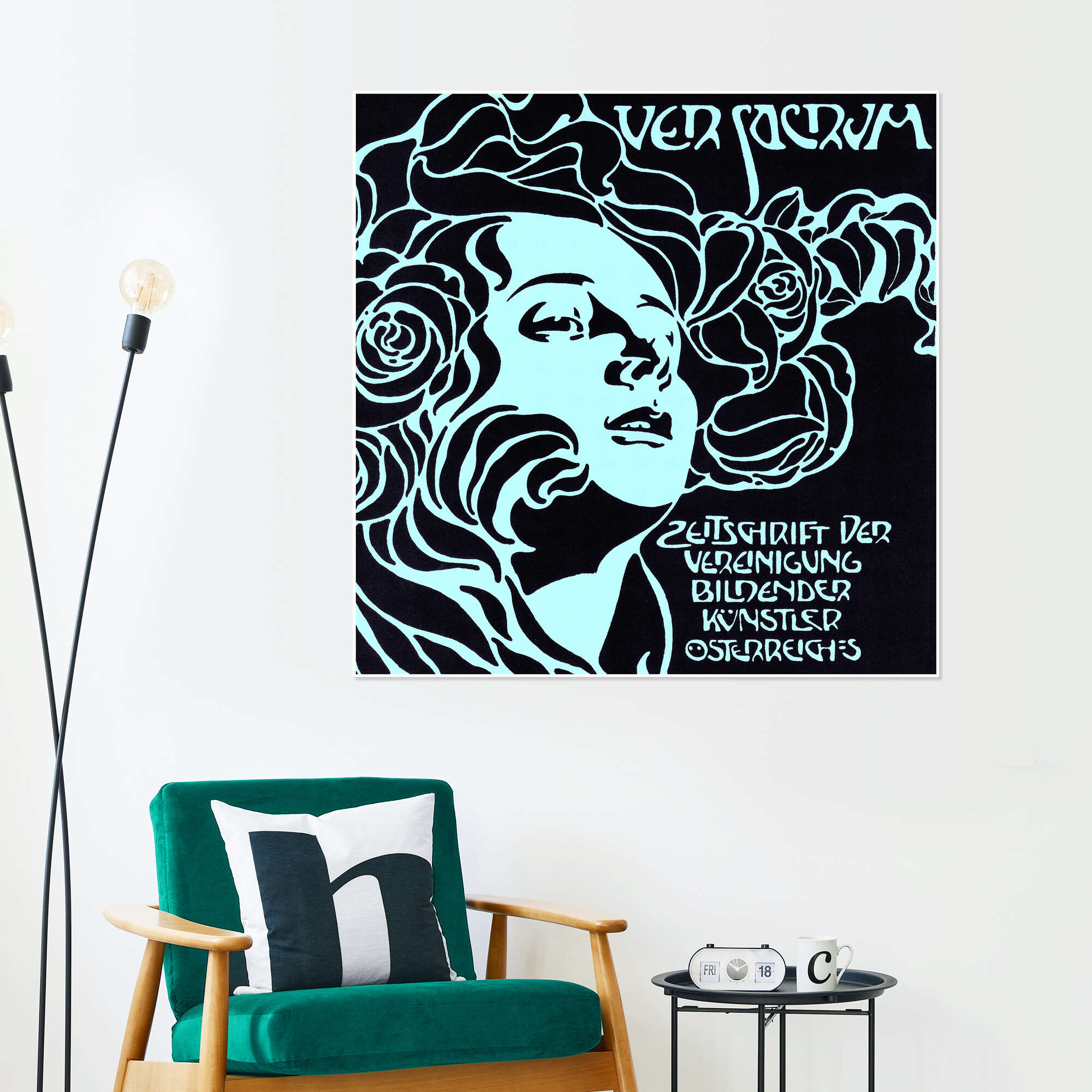This image captures a meticulously arranged room setup that appears to be part of an advertising photo or a design showcase. Dominating the scene is a large, black poster on the wall featuring a stylized drawing of a woman's face in light aqua, her hair adorned with abstract roses, and text in German. Below the poster sits a chic, wooden easy chair with open arms, its cushions upholstered in dark green, soft material. The chair is accented by a white throw pillow bearing a capital letter 'H' in a contrasting color, possibly black or dark green.

Flanking the chair is a modern floor lamp with an X-pattern design and two exposed bulbs pointing upwards from slender, long black stems. To the other side of the chair, a sleek black side table with four legs and a circular top holds a small analog alarm clock displaying 'Friday the 18th' and nearly 2 o’clock. Next to the clock is a white coffee mug with a black capital letter 'C' printed on it. The overall arrangement combines contemporary elements with a touch of artistic flair, emphasizing the cohesion of modern design and comfort.